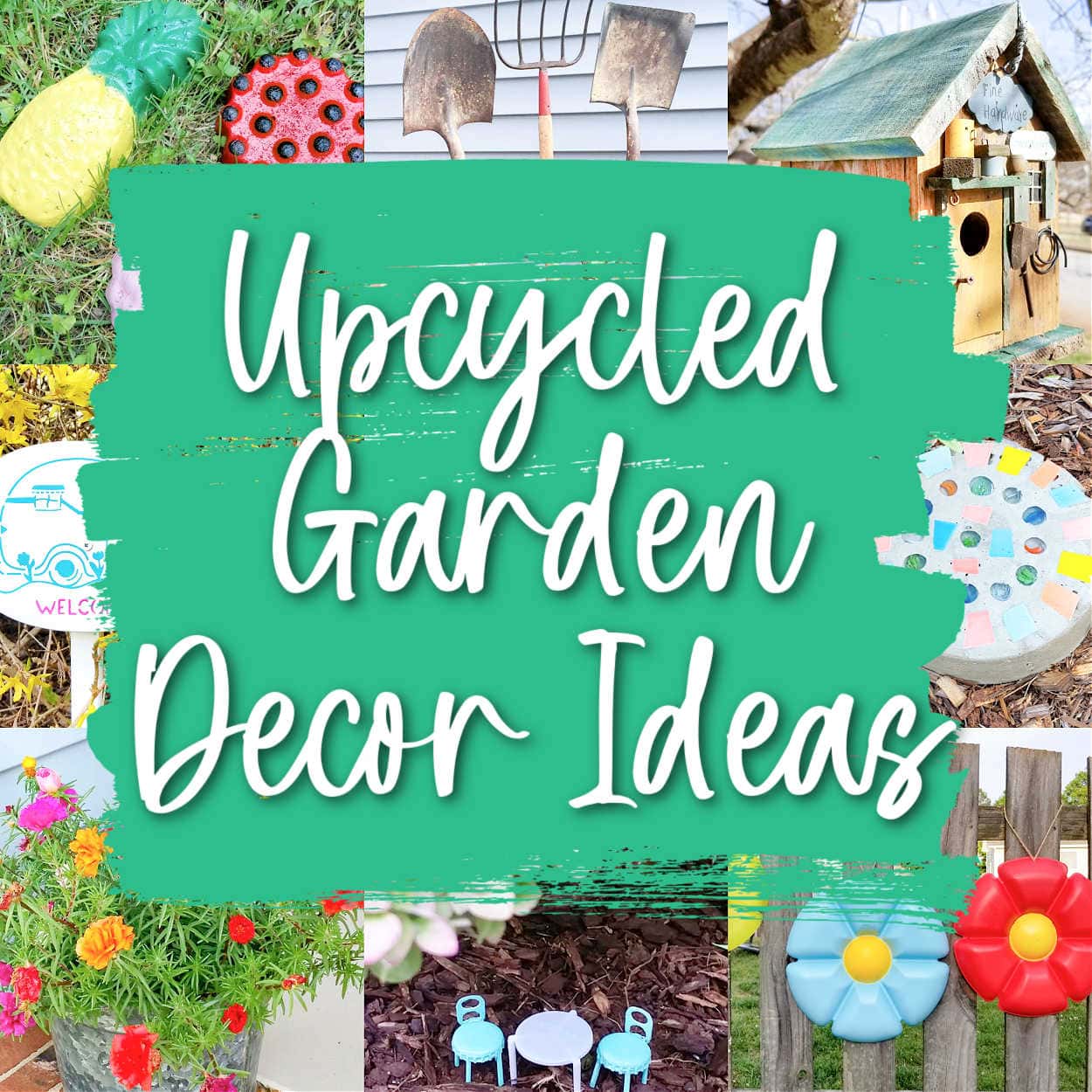The image is a visually rich collage of eight garden-themed photographs arranged around the perimeter and overlayed with central text and graphics. The photographs depict various elements typically found in a garden, including whimsical lawn decorations, a quaint wooden shed, a flowering bush in a metal pot, and a vibrant flower planter brimming with red and pink blooms. The images also show colorful garden furniture, a purple table paired with light blue chairs, and creatively upcycled items like a plastic pineapple and decorative flowers crafted from plastic in light blue and red with yellow centers. Intersection points in the image feature crucial garden tools such as shovels and a pitchfork, while the top right corner showcases a handcrafted birdhouse. Dominating the center of the collage is a bold green background marked with three paint-like stripes, over which elegant white cursive text reads "Upcycled Garden Decor Ideas" in three lines. This central text pulls together the various visual elements, highlighting the theme of innovative garden decor using upcycled materials.